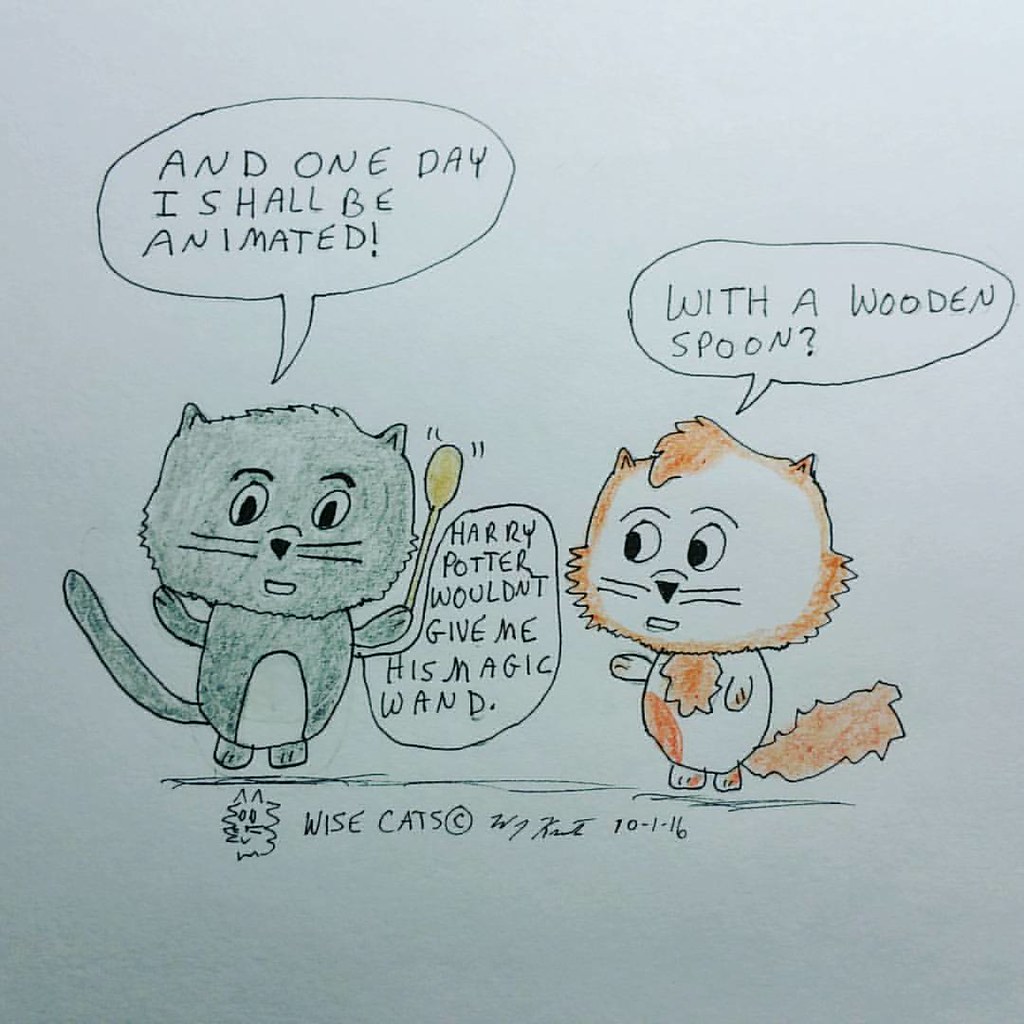This is a photograph of a hand-drawn cartoon in pen and ink, depicting a humorous interaction between two anthropomorphic cats with exaggerated features, including large heads and big eyes. The gray cat on the left, holding a wooden spoon with animated movement indicated by its raised tail, boldly declares, "And one day I shall be animated." This cat is looking at the viewer while waving the spoon. The orange cat on the right, marked with yellowish-orange spots, faces the gray cat and responds with skepticism, saying, "With a wooden spoon?" The gray cat then retorts, "Harry Potter wouldn't give me his magic wand." At the bottom of the illustration, there's a small sketch of a smiling cat face, accompanied by the text "Wise Cat's Copyright" and the artist's signature dated 10-1-16.